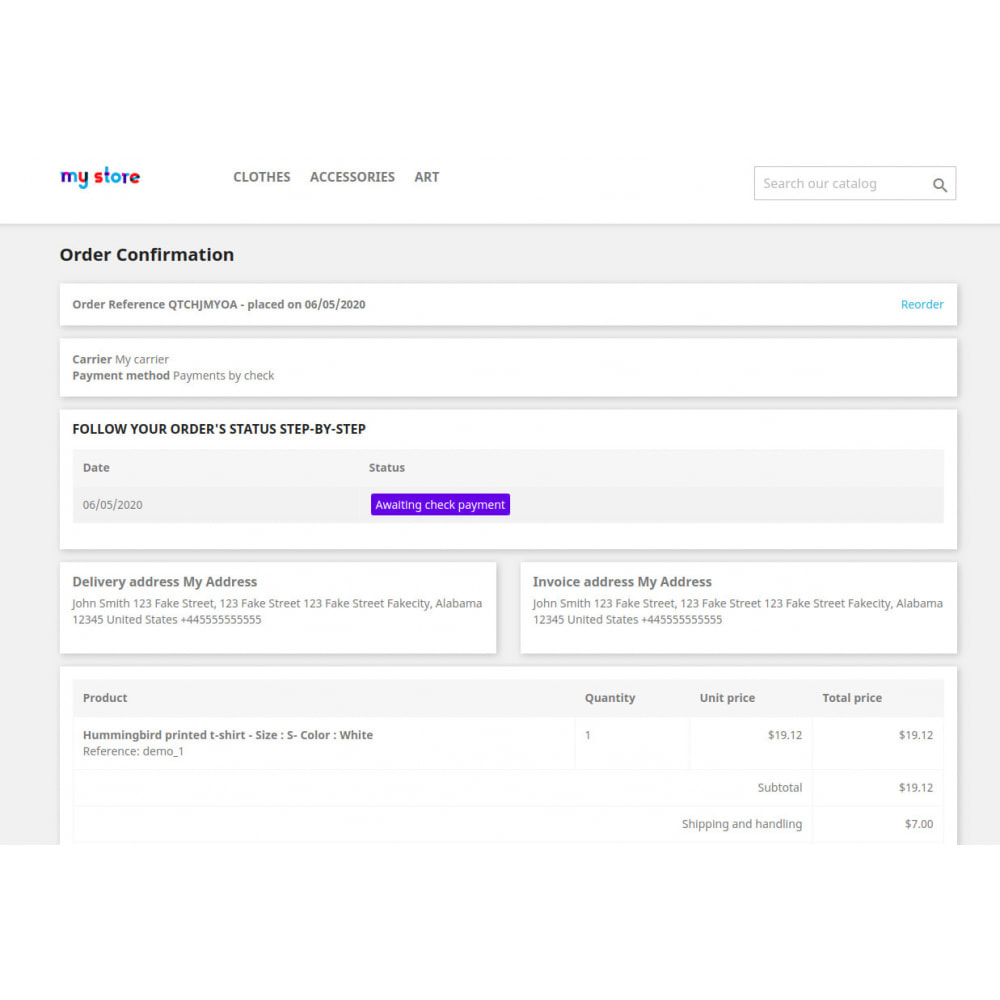The image depicts a colorful and vibrant website for a company named "MyStore" (spelled M-Y-S-T-O-R-E), with each letter in a different hue: purple, red, green, red, blue, blue, purple. At the top, the website highlights that it sells clothes, accessories, and art. Featured prominently is a search bar.

In a gray section, there's a heading in dark black lettering that reads "Order Confirmation." Within this section, a white strip details the order reference number, with a prompt showing the order was placed on April 5, 2020. There's also a blue button at the end labeled "Reorder" for easy reordering.

Another separate section outlines the carrier and payment method, indicating that the payment was made by check. Further down, a third section titled "Follow Your Order Status" offers a step-by-step update on the order. It mentions the date of the order and the status, which currently is "Awaiting Check Payment."

Following that, there are sections confirming the delivery and invoice addresses, both reflecting the purchaser’s address. The final section, "Product Information," lists the ordered item: a Hummingbird Printed T-shirt, size Small, color White, with one unit purchased. The unit price is stated as $19.12, making the total product cost $19.12. Additional charges for shipping and handling are $7.00, although the full price of the order isn't visible.